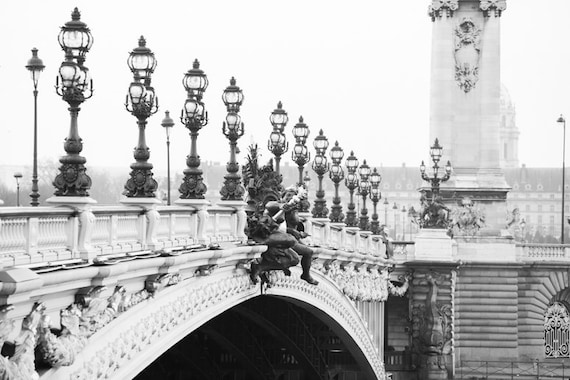This black-and-white photograph captures an ornate European bridge, possibly located in the UK or France. The bridge, crafted from white stone, features elegant railings with intricately designed lampposts at regular intervals, each adorned with two spherical bulbs. A closer look reveals a series of statues along the railing, one of which appears vaguely humanoid, perched upon the edge. The bridge likely spans a waterway, as suggested by the dark, obscured space beneath it.

On the far side, a variety of slender, single-bulbed lampposts continue the illumination. A grand architectural structure with a prominent spire rises in the background, adding to the majestic atmosphere of the scene. The bridge’s sophisticated design and surrounding elements, such as a towering column and detailed carvings, enhance its prestigious and historical appeal. The entire image, rendered in shades of black, white, and gray, exudes an air of historical significance and timeless elegance.